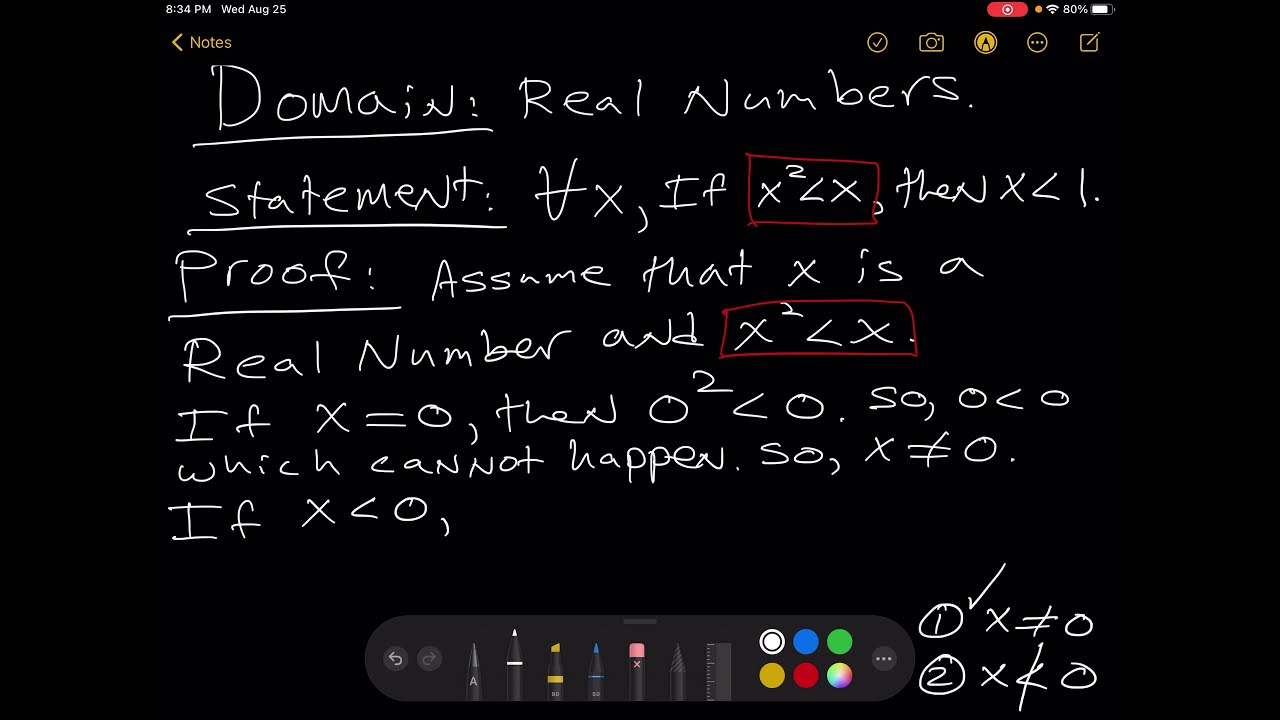This horizontal rectangular image, captured on an Apple device, features a handwriting-styled note on a black background. At the top left, the screen shows the time as 8:34 p.m. on Wednesday, August 25th, while the top right displays icons for screen recording, Wi-Fi signal, and an 80% battery indicator. The note is organized with several handwritten sections, all left-aligned in white ink.

The note begins with "Domain:" underlined, followed by "real numbers." Directly below, "Statement:" is also underlined, with "∀X, if X² < X (circled in red), then X < 1." proceeding it. Further down, "Proof:" is underlined and delineated into several steps:

1. "Assume that X is a real number and X² < X" (also circled in red).
2. "If X = 0, then 0² < 0 so 0 < 0, which cannot happen. Therefore, X ≠ 0."
3. "If X < 0..." (incomplete).

In the lower right corner, sequential steps are marked: "1" circled with a checkmark next to "X ≠ 0," followed by "2" with "X < 0" crossed out, indicating an error.

The bottom-center of the screen displays an elongated oval shape containing icons for various digital pens and color palettes, offering options in white, blue, green, yellow, red, and gray for note-taking.